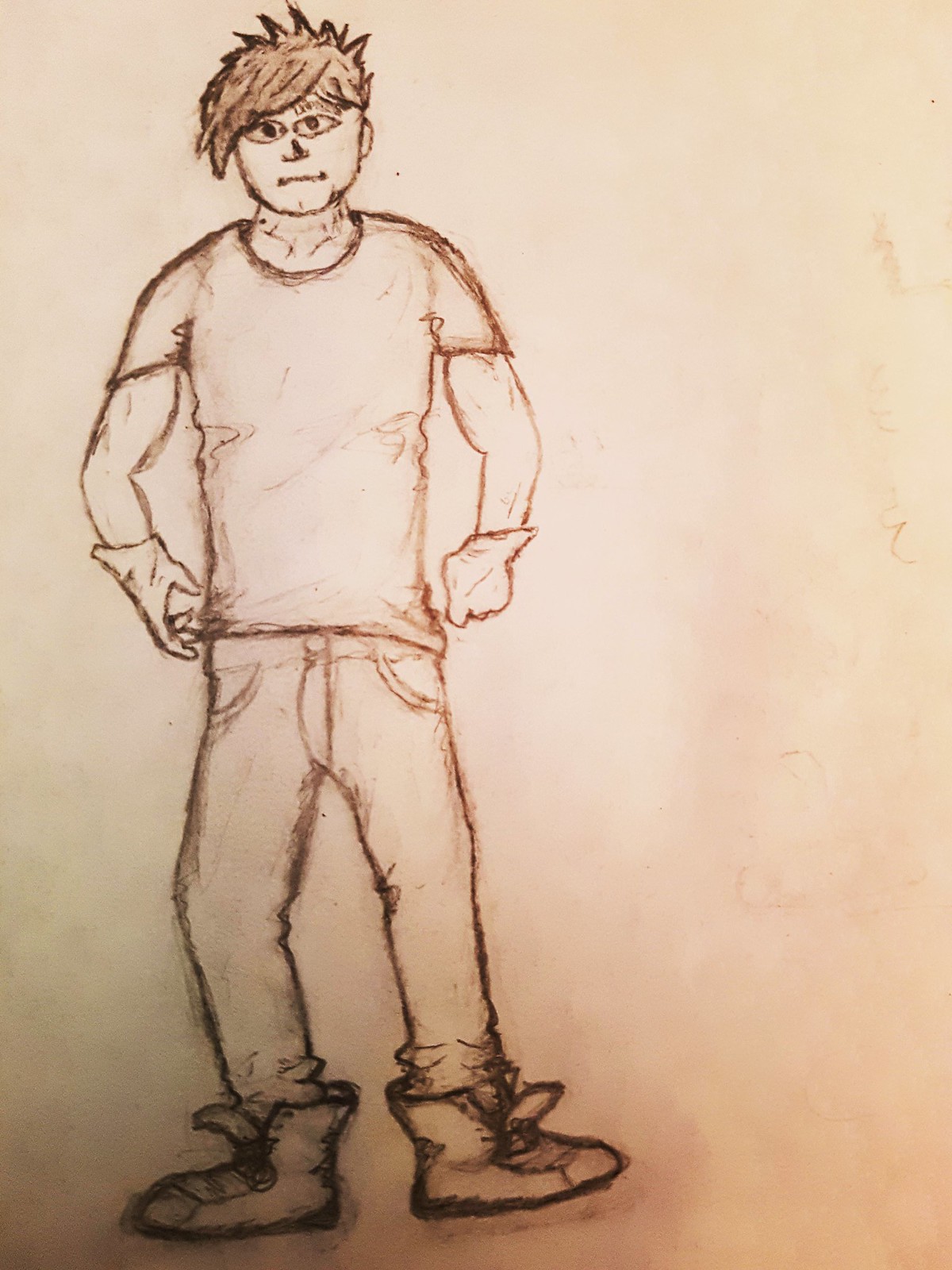This is an illustration created on light brown-colored paper, seemingly by a child or teenager. The artwork features a young man positioned to the left side of the page, rendered in brown pencils. The character is depicted in an anime or manga style, characterized by large, expressive eyes. He has spiky brown hair that cascades in waves over his forehead. His facial features include a small nose and a thin, horizontal line for a mouth. The young man is dressed in a short-sleeved shirt and gloves, paired with jeans. His outfit is completed with boots, which are notably detailed with tongues flopping over and unlaced at the top. The drawing contains no accompanying text or inscriptions.